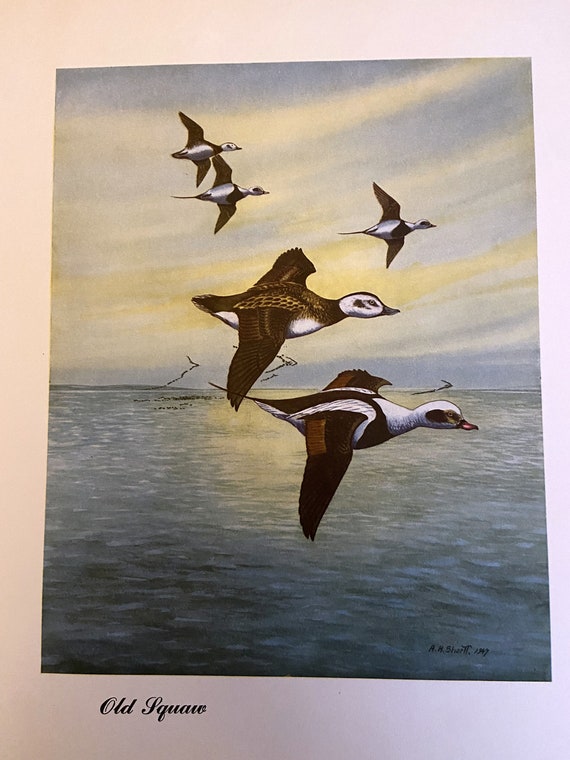This image depicts a painting centered within a white postcard-sized border. The bottom left corner of the white backing features the cursive inscription "Old Square." The painted scene showcases five birds in mid-flight above a shimmering expanse of ocean. The birds, identified by their distinctive white heads and primarily dark wings, convoke a serene twilight ambiance, evident from the sky's gradient of blue and gold hues with streaks of gray.

In the foreground, two birds appear close to the viewer, showcasing slightly varied patterns—the nearer one sporting more white on its body. Behind them, three additional birds trail in the distance, arranged dynamically in the composition. Subtle indications in the farthest background hint at other avian forms, though these are more abstract and less detailed.

The sky, donned in soft yellow streaks against a blue backdrop, and the reflective gold tones in the water further emphasize the twilight setting. The ocean exhibits reflections of the distant sun, enhancing the painting's tranquil and almost ethereal quality. The artist's signature and date are delicately placed in the bottom right corner of the painting, enunciating the creator's final touch to this evocative scene.